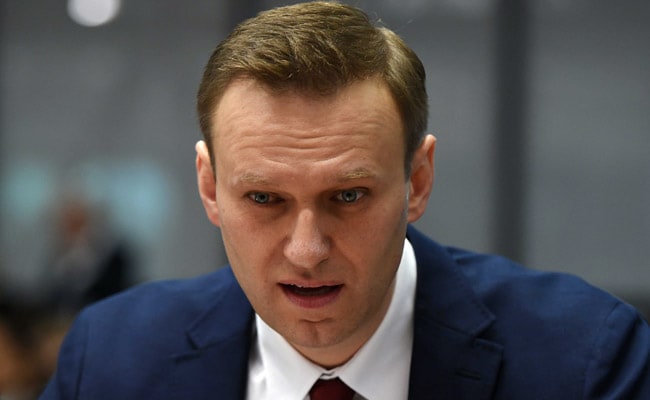The image showcases a close-up of a serious-looking man dressed in a navy blue suit jacket, a white button-up shirt with a collar, and a burgundy tie. His expression is one of concern, with furrows on his forehead and a slightly open mouth, suggesting he might be in the middle of talking or deeply focused on reading something. His brownish-blonde hair is neatly parted to the side and combed back slightly at the front, complementing his light blonde eyebrows and blue eyes. The photograph, set against a blurred gray background, appears to be taken indoors with suboptimal lighting, contributing to the image's relatively noisy and poor quality. The man, who is clean-shaven and around 40 years old, gives off an air of professionalism, possibly hinting at a role such as a lawyer, businessman, or politician.